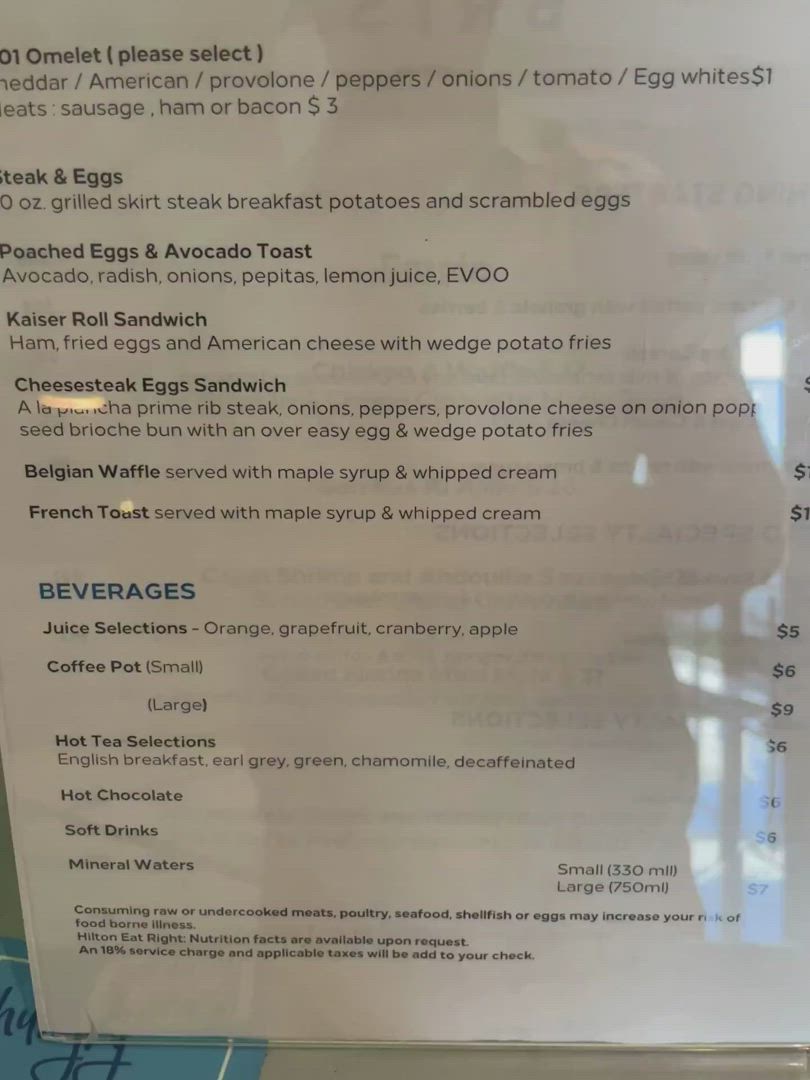This image features a classic American diner menu, meticulously laminated in clear plastic to prevent damage. The menu is large and well-organized, starting with a section dedicated to a variety of omelettes. Diners can customize their omelettes with a selection of cheeses—Cheddar, American, and Provolone—as well as vegetables like peppers, onions, and tomatoes. Egg whites are available for an additional dollar, and meat options such as sausage, ham, or bacon can be added for three dollars.

The next entrée listed is steak and eggs, followed by poached eggs with avocado toast. Other breakfast specialties include a Kaiser roll sandwich, cheese steak egg sandwich, and a Belgian waffle. The Belgian waffle section notes that it comes with maple syrup and whipped cream, giving diners a complete and indulgent breakfast experience.

Further down, the menu offers French toast, again served with maple syrup and whipped cream. The beverage section includes an array of juice options such as orange, grapefruit, cranberry, and apple. Coffee is available in small or large pots, and there's a selection of hot teas, hot chocolate, soft drinks, and mineral waters.

The bottom of the menu contains some additional writing, possibly detailing restaurant policies, extra items, or promotional information.